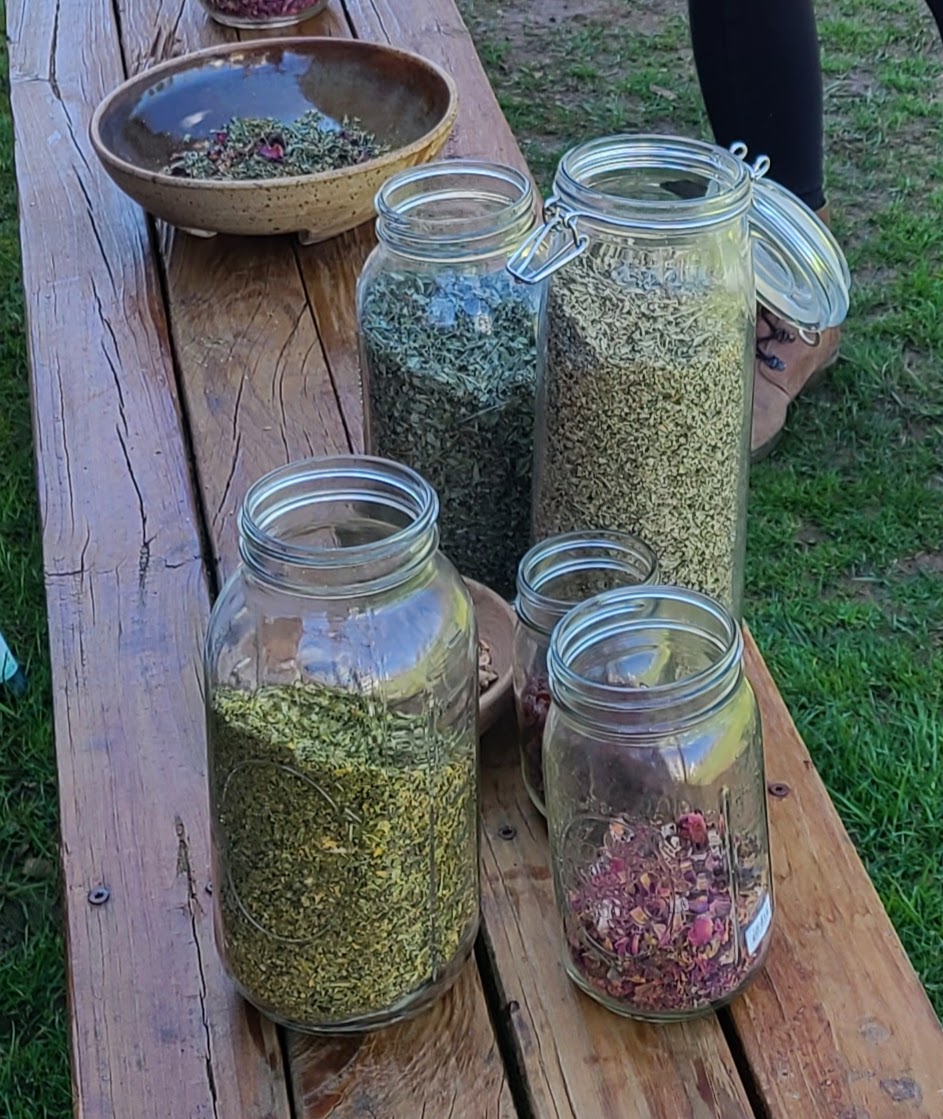The image depicts a tranquil outdoor scene with a green grass background and a rustic wooden bench stretching from the upper left corner to nearly the bottom right of the frame. The bench is comprised of four wooden slats and holds an assortment of glass jars and bowls. There are six jars in varying sizes filled with dried herbs of different shades; the tallest jar, almost full, contains sage green herbs, while a darker green herb is in the jar next to it. Among the jars, one displays a grass-green herb and another in the foreground holds purple herbs, with one jar partially obscured. Nestled between the jars is a smaller bowl, and further back to the upper left, a shiny brown bowl contains a mixture of dried green and reddish-purple herbs. At the upper right, partially out of focus, a person's leg dressed in black pants with a brown shoe can be seen behind the tallest jar. The overall scene suggests a laid-back atmosphere, possibly late in the day, with the jars likely used for storing dried herbs or spices, potentially for cooking or brewing purposes.